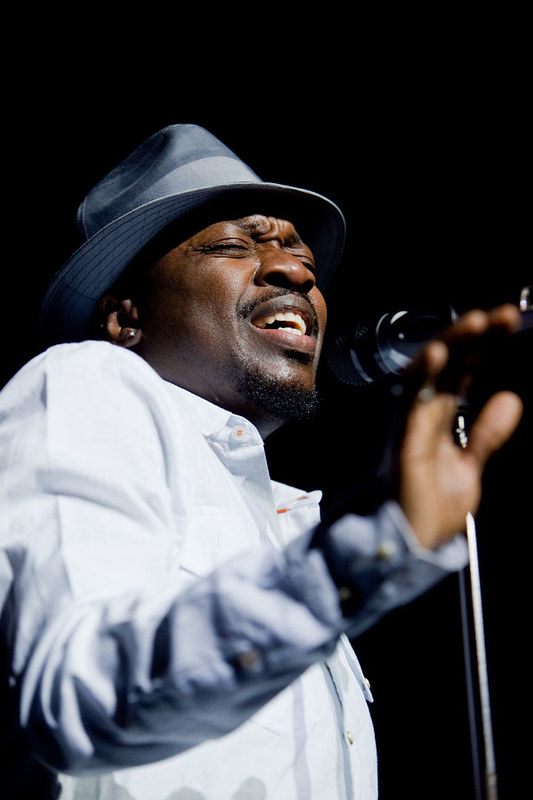The image captures an intense moment of a nighttime concert, featuring a black male singer deeply immersed in his performance. With his eyes closed and mouth open, the singer's emotional connection to the music is palpable. He stands in front of a microphone mounted on a freestanding metal stand, with the black microphone's mesh design clearly visible. The singer sports a thin black mustache and a small goatee. Adorning his head is a gray or silver metallic hat, possibly a fedora, which has a patterned inner brim. He wears a simple white dress shirt with clear, opaque buttons, sewn on with distinctive orange thread. An earring gleams in his right ear, further highlighting his expressive demeanor. The background is pitch black, suggesting a concert at night, with a bright light illuminating him, making him shine against the dark backdrop. His raised hand adds to the sense of rhythm and passion that he brings to this powerful performance moment.